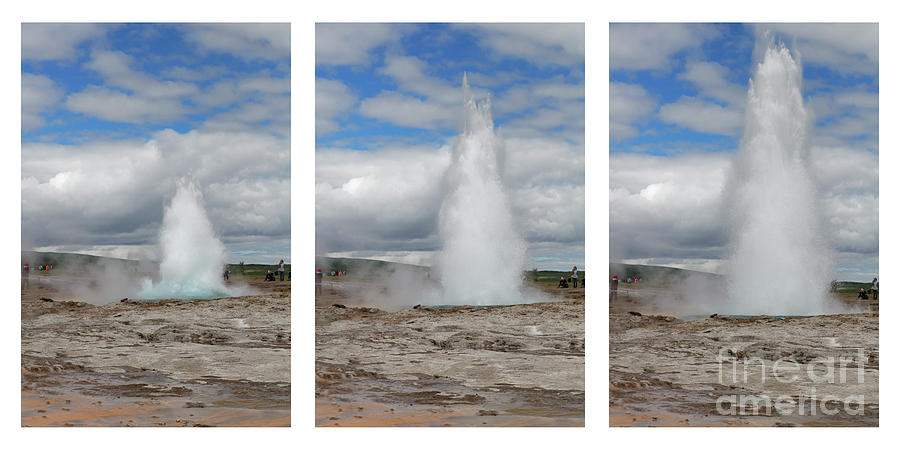The image is a three-panel fine art photograph from "Fine Art America," depicting a geyser in different stages of eruption. Each of the rectangular panels captures the geyser at a distinct phase: the left panel shows the initial burst with a small plume of steam, the middle panel captures a more pronounced eruption, and the right panel illustrates the geyser at its peak, with steam reaching the top of the image. Set against a vivid blue sky adorned with white and gray clouds, the surrounding environment features a dusty dirt ground with shades of rust orange in the bottom left corners of each photo, and rolling hills in the background. The geyser's plume is a striking white, while the base shows hints of light blue water. In the bottom right corner of the image, there is a faint white watermark that reads "Fine Art America." The overall composition, likely taken in a place known for such natural spectacles, beautifully showcases the geyser's dynamic eruption stages.